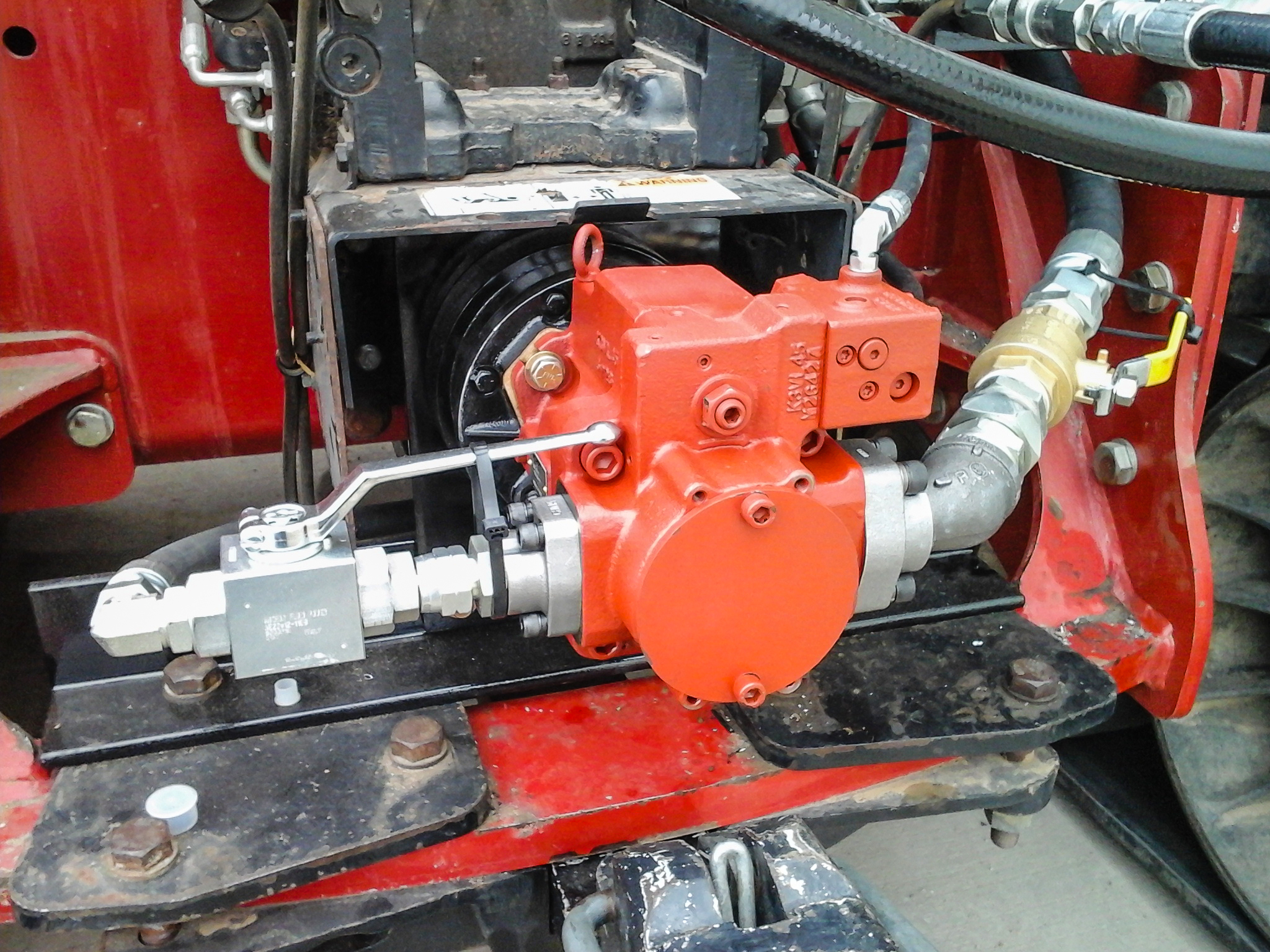The image is a close-up of the inner workings of a machinery, prominently featuring a bright orange engine part at the center. This central component has metallic tubes coming off each side, and black hoses are attached to various sections of it. In the background, a vehicle painted in bright red is visible, with three bolts on the left and one on the right securing parts of it. The upper right corner of the image shows engraved but unreadable lettering on the orange part. Additionally, there is black tubing in the top right corner and a hint of a wheel just visible at the very edge of the frame. The setting seems to be inside a red casing, possibly indicating that this machinery could be part of farm equipment or an automobile undergoing maintenance, with multiple smaller hoses, which may include electrical components, surrounding the main engine.